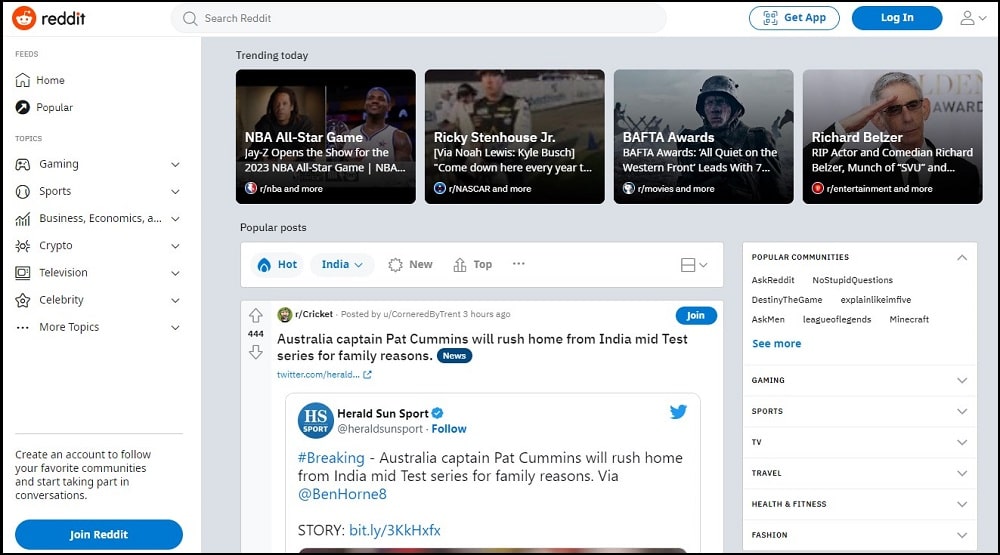Screenshot of the Reddit Website:

This screenshot captures the main interface of the Reddit website. In the upper-left corner, there's a distinctive circular, orangish-red icon featuring the face of Reddit's mascot, which resembles an alien or robot. This character is white with an antenna protruding from the top of its head. Immediately to the right of this icon is the Reddit name.

Centrally placed in the image, there's a long, rectangular search bar with curved edges, colored in light gray. Moving to the upper right corner, there are two prominent buttons. One is outlined in blue with blue text reading "Get App," and the other has a dark blue background with white text stating "Log In." Further right, there's a gray user icon accompanied by a downward-facing arrow, likely indicating a menu for user options.

Below this top navigation bar, there are four trending articles, each with its own image. These images are rectangular and depict various individuals in different costumes, likely representing athletes and actors. The titles of these articles are written in white text overlaying the images.

Further down, in the section for popular posts, there's a highlighted post that has garnered 444 likes. The entire background of the screenshot is light gray, with several sections featuring square and rectangular shapes with white backgrounds. Additionally, on the left side of the image, there's a menu with a white background and dark gray text, providing easy navigation through different sections of the site.